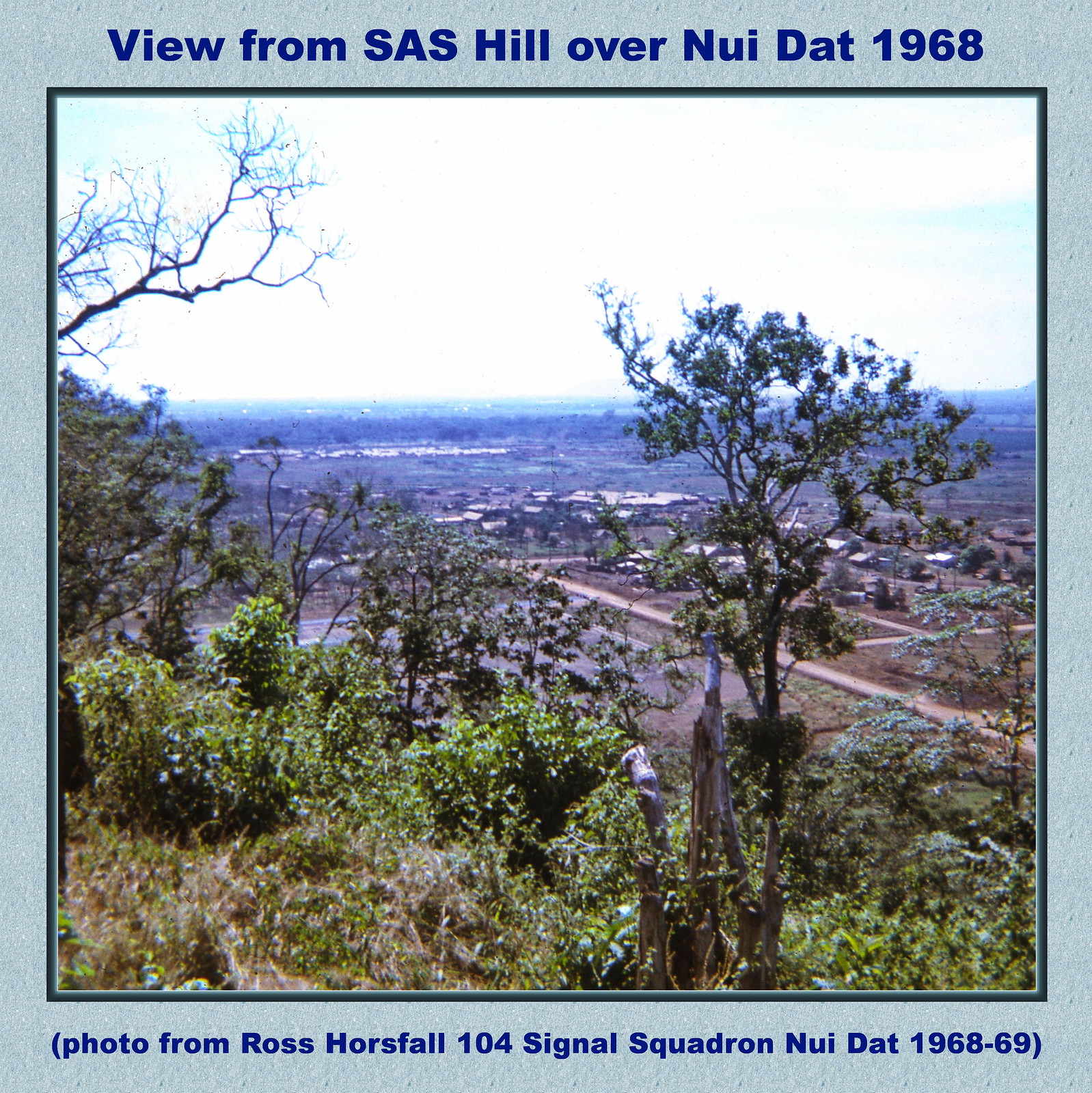This photograph captures an expansive landscape viewed from the top of SAS Hill over Nui Dat in 1968. The foreground is rich with greenery including bushes, weeds, grasses, and scattered flowering plants, while the mid-ground shows a sparser collection of trees with small leaves, some appearing to be dried and losing their lushness. The land stretches out into a flat, broad valley characterized by predominantly brown and dry grasses, indicating a somewhat arid environment. Stitched into this landscape are the distant, modest structures of a sparsely populated village, their small size making the area appear somewhat desolate. Despite the sparse population visible, there are scattered buildings far off in the distance nestled among the plains and trees. The sky above is clear, but the horizon is overly bright, almost blown out with a light blue hue. Surrounding the image is a gray border with text: at the top in light blue letters, it reads “View from SAS Hill over Nui Dat, 1968.” At the bottom, in parentheses, it says, “Photo from Ross Horsefall, 104 Signal Squadron, Nui Dat, 1968-1969.”